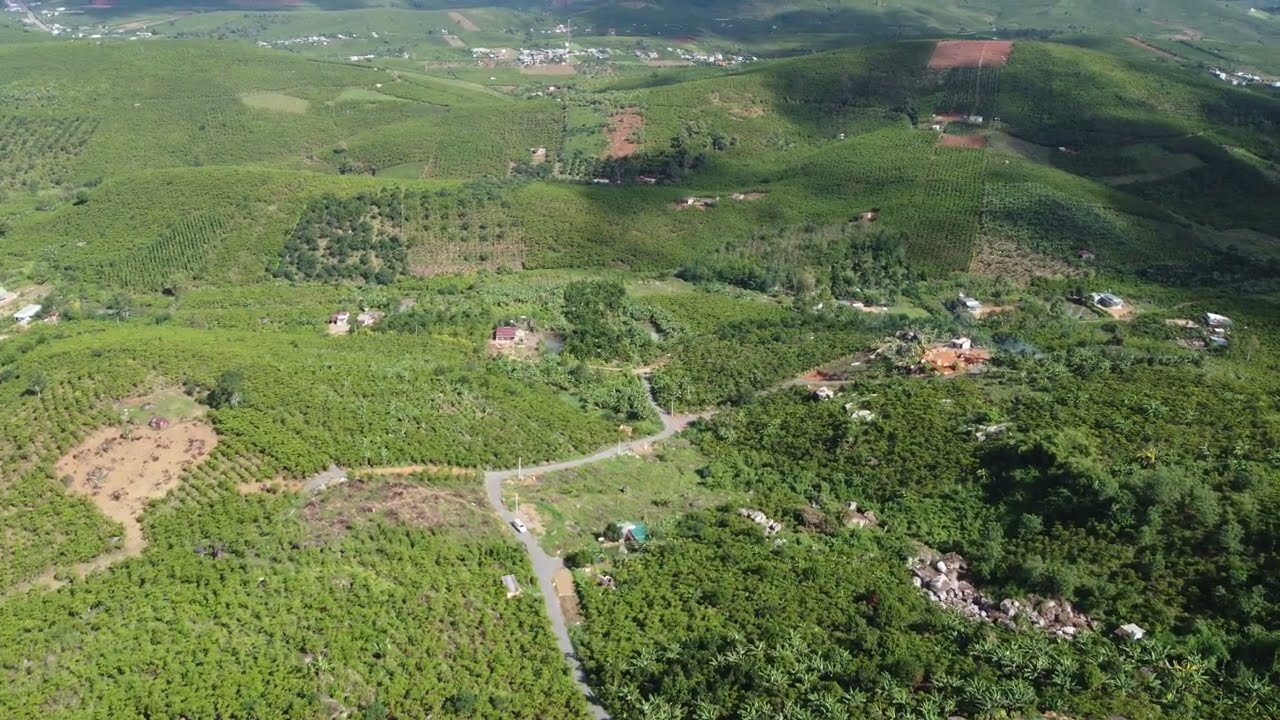This is an aerial photograph taken during the daytime, capturing a rural landscape featuring farmland with rolling hills. The top-right corner of the image shows these hills with shadows cast by unseen clouds above, creating contrasting darker patches amidst the vibrant greenery. Scattered across the hills are rows of trees or bushes, likely forming grapevines or similar agricultural arrangements. In addition to the rolling terrain, the image includes various neatly tilled fields, predominantly brown, interspersed throughout the landscape.

In the lower right-hand corner, rocky outcroppings and possibly small houses or buildings are visible, appearing almost like beehives due to the high elevation from which the photograph is taken. A narrow road starts from the center bottom of the image, winding its way upward before sharply bending to the right and eventually branching out across the hills towards the upper right. The left side of the hills is densely populated with trees and lush vegetation.

Colors in the scene range from the rich browns of tilled earth to the various shades of green in the foliage, accented by touches of white, gray, and black from the scattered houses, rocks, and roads. The view encapsulates the essence of rural farmland, with its intricate mix of natural and cultivated features, all presented under the clear light of a sunny day.